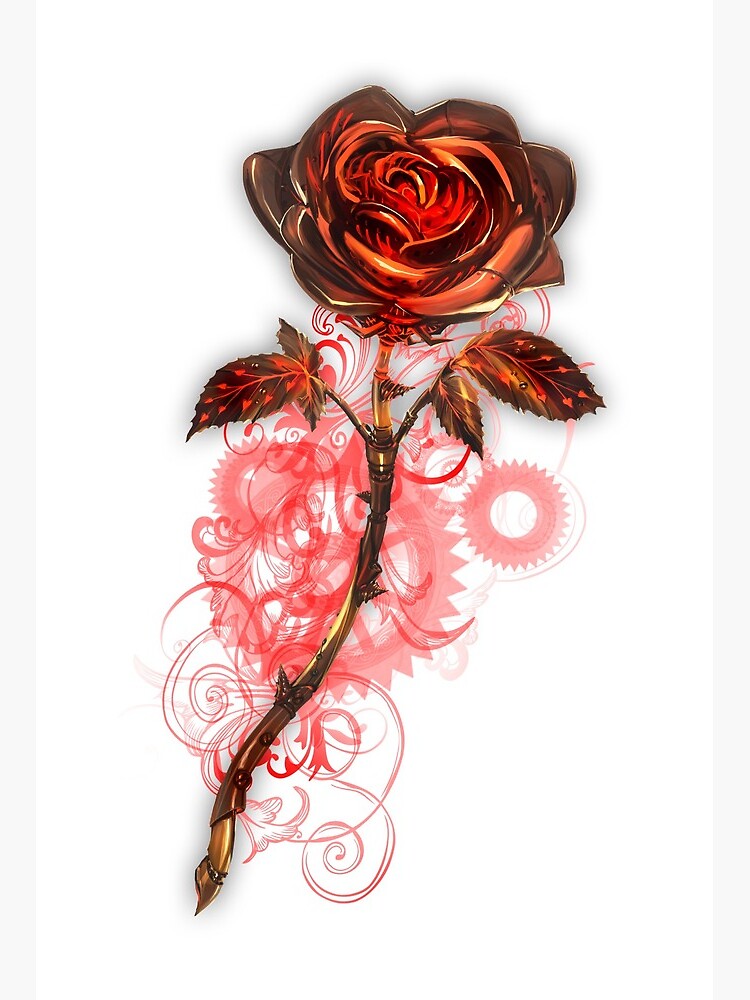This image is a computer-generated, 3D-illustration of a rose with a detailed, metallic appearance. The rose features a striking contrast between its brightly colored red interior petals and dark brown exterior petals, accented with a metallic, possibly copper or brass, tint. The stem, rendered in a gold or copper hue, appears intricate and wiry, extending to equally detailed leaves that combine gold tones with small, spiky red dots. Beneath and around the rose, there are cogwheel shapes, resembling spur gears, intertwined with transparent red swirls and floral patterns. The entire composition is set against a white background, enhancing the clarity and vibrancy of the rose and its elaborate mechanical and artistic elements.